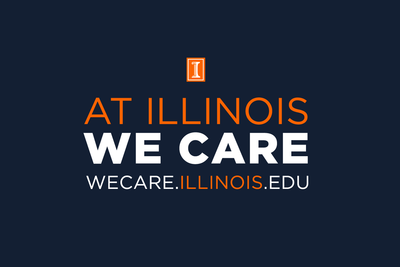This detailed caption describes an image of what seems to be a homepage or poster for the website "wecare.illinois.edu":

---

The image displays what appears to be either a webpage or a poster for the website "wecare.illinois.edu." The background of the page is a dark blue color. Prominently featured is an icon consisting of an uppercase letter 'I' in varying shades of orange and white, enclosed within an orange square. Below the icon is the text "At Illinois, we care," with "At Illinois" rendered in orange and "we care" in white. At the bottom of the image, the URL for the website, "wecare.illinois.edu," is clearly listed. There are no visible tabs or navigation elements, suggesting that this may indeed be a poster rather than a webpage.

---